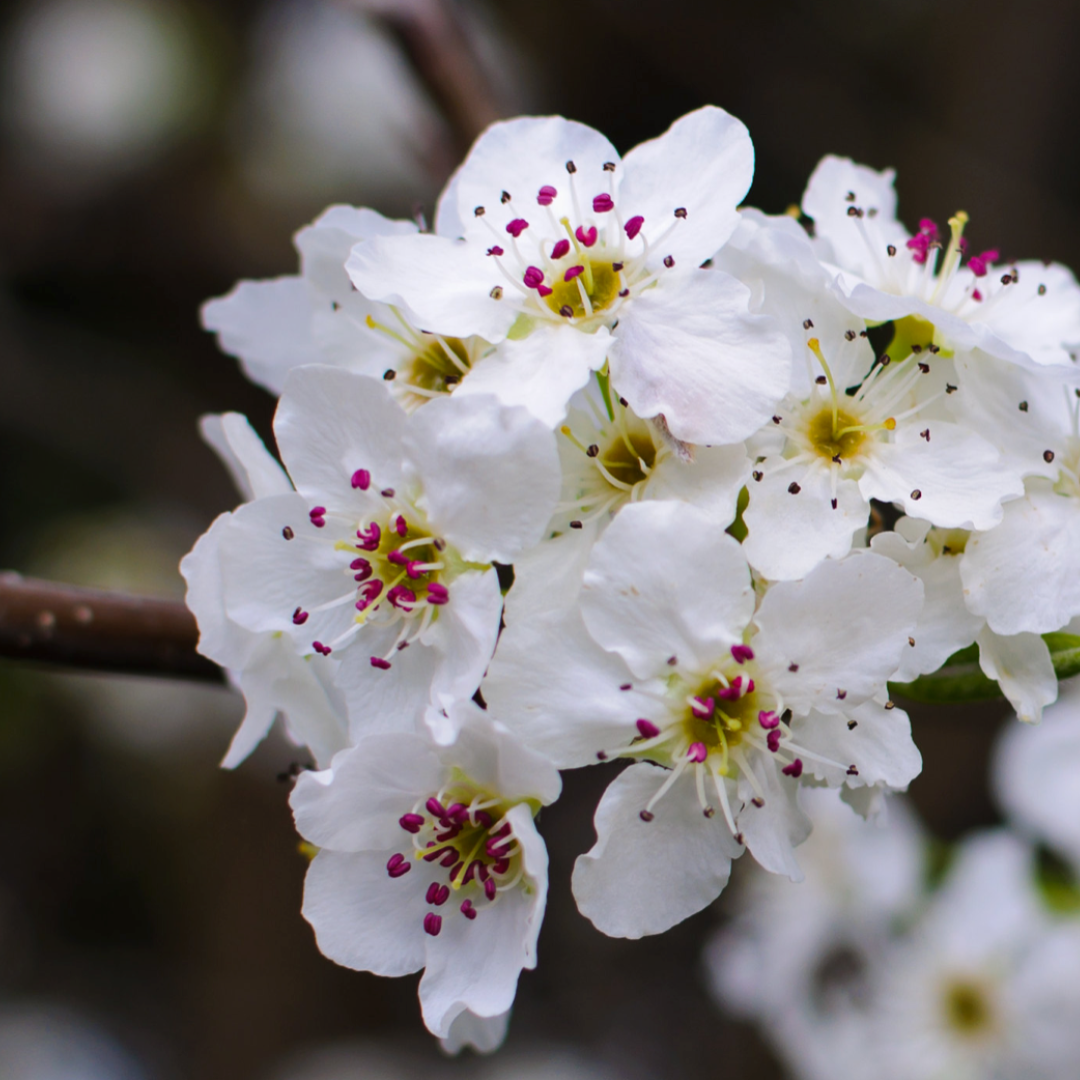This photograph is a close-up view of a cluster of beautiful white flowers, each featuring five delicate petals. The stamens of these flowers vary in appearance: some have tiny, rose-colored tips while others exhibit vibrant pink tops, all centered around a muted yellow core. The focal point of the image is on approximately ten flowers blooming on a single stem, which can be seen towards the center left of the composition. The background is elegantly blurred, creating a stark contrast with the dark black areas on both the right and left sides, lightly highlighted by blurred white shapes that suggest additional flowers. This zoomed-in photo meticulously captures the natural elegance of these flowers, perfect for use in scientific publications or magazines.